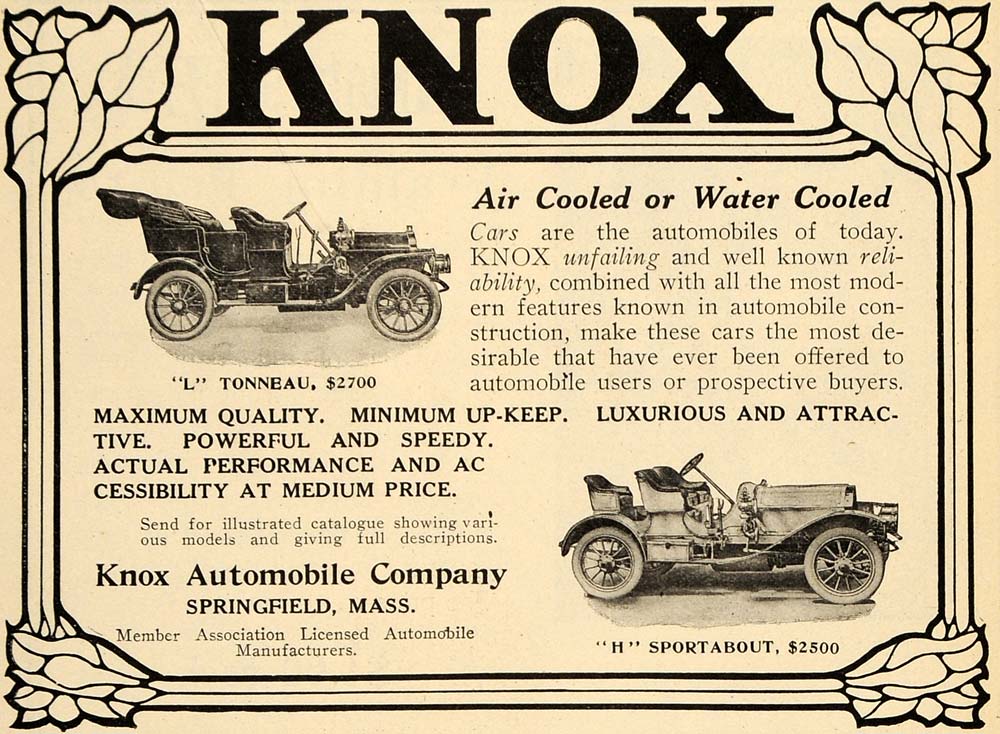The image is a vintage advertisement, likely from the early 20th century, printed on old beige or off-white paper with a decorative border featuring leaves in each corner. Dominating the top of the advertisement in bold black letters is the name "KNOX." Below this, the ad showcases two antique automobiles, mentioned for their air-cooled and water-cooled features and priced at $2,700 and $2,500. The text emphasizes Knox’s unfailing and well-known reliability, combined with all the modern features of the time, making these cars the most desirable for automobile users and prospective buyers. The description highlights these vehicles as luxurious, attractive, powerful, and speedy, with maximum quality and minimum upkeep, effectively offering actual performance and accessibility at a medium price. The advertisement concludes with an invitation to send for illustrated catalogs displaying various models and providing full descriptions. The ad is from the Knox Automobile Company, based in Springfield, Massachusetts, and notes its membership in the Association of Licensed Automobile Manufacturers.